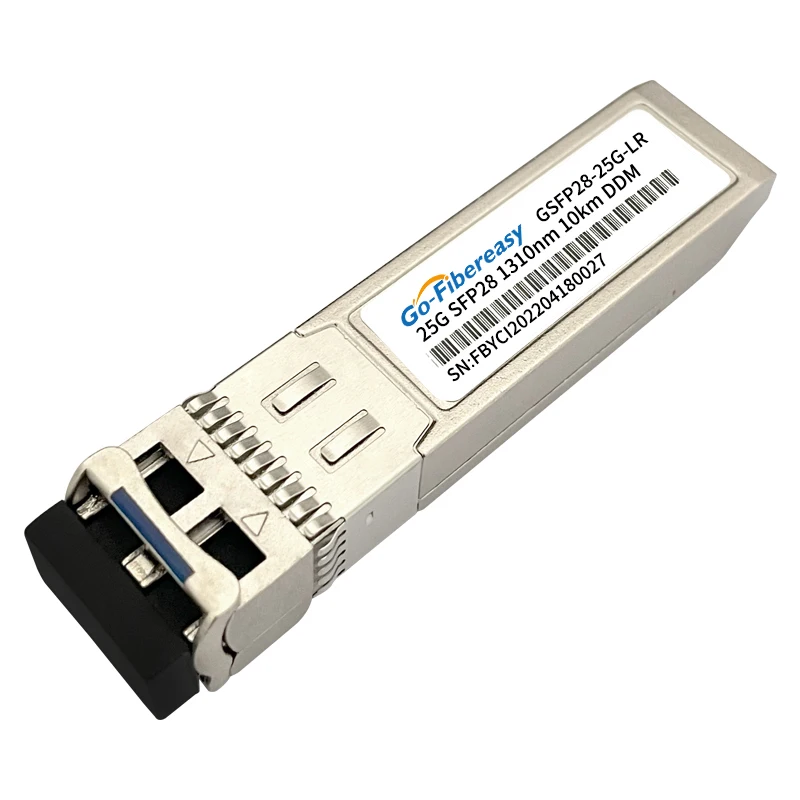The image displays a close-up, detailed photograph of a long, rectangular gray object, diagonally positioned against a white background, spanning from the upper right to the lower left corner. The top side of the object features a white label with blue text, reading "Go Fiber Easy" underneath a yellow arc. Below this, it displays alphanumeric codes "GSFP28-25G-LR," "25GSFP28," "1310NM," and "10KMDDM." Further down, there's a barcode accompanied by another string of characters: "SN: FBYC1202204180027." On the left side of the object, there is a black rectangular attachment. The purpose of the object is unclear, and it could range from a small office tool to a larger electronic component.